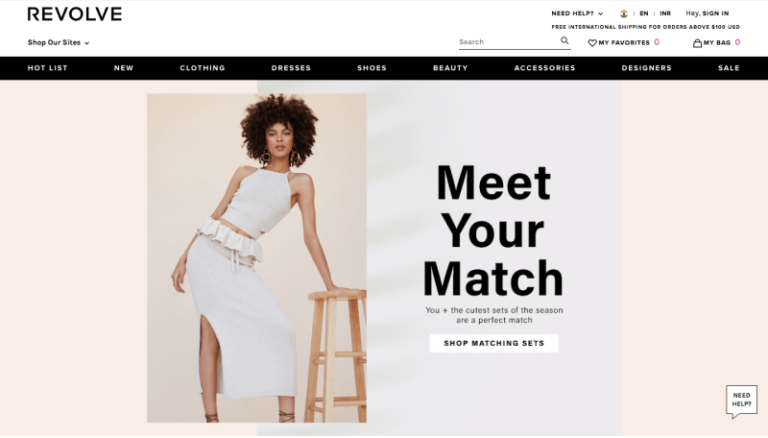The image depicts a sleek webpage for a brand called "Revoltal," prominently displayed in the top-left corner with its name spelled out as "R-E-V-O-L-T-A-L." Directly beneath the logo, the text "Shop Our Sites" invites users to explore further. Below this header, a navigation bar stretches horizontally with tabs labeled: Hauntless, New, Clothing, Dresses, Shoes, Beauty, Accessories, Designers, and Sales, providing a comprehensive menu for potential shoppers.

Central to the webpage is a striking photograph of a woman standing confidently. She has voluminous brown hair and is stylishly dressed in an all-white ensemble, featuring a sleeveless top and matching bottoms. Her left hand rests lightly on a stool placed to the right side of the image. The backdrop is a minimalist gray, keeping the focus on the subject and her attire.

To the right of the image, bold text reads "Meet Your Match," suggesting a perfect pairing between the viewer and the season's most attractive sets. A call-to-action button below urges users to "Shop Matching Sets." In the bottom-right corner of the page, a helpful prompt questions, "Need Help?" presumably linking to customer support resources.